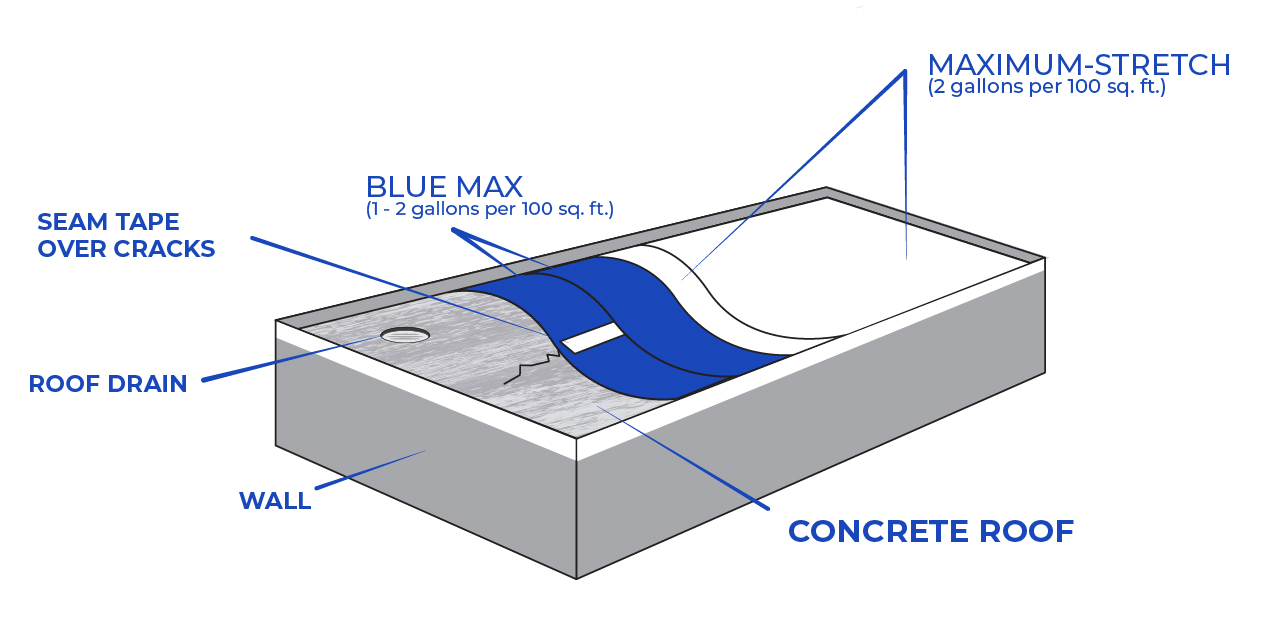The diagram features a grey rectangular box oriented at an angle from the bottom left to top right. The box has a white outline around its top edge. Within this box, there is an inset section viewed from above, with a mottled grey background on the left side that includes a hole labeled "Roof Drain" and a crack labeled "Seam Tape Over Cracks." Adjacent to the cracked area are two solid blue waves labeled "Blue Max" with the note "(1-2 gallons per 100 square feet)." Next to these blue waves is a solid white wave, followed by the rest of the inset section filled with pure white, labeled "Maximum Stretch" with the note "(2 gallons per 100 square feet)." Blue text and lines point to various parts of the box: the entirety of the mottled grey area is labeled "Concrete Roof," and the main outside portion of the box is labeled "Wall."